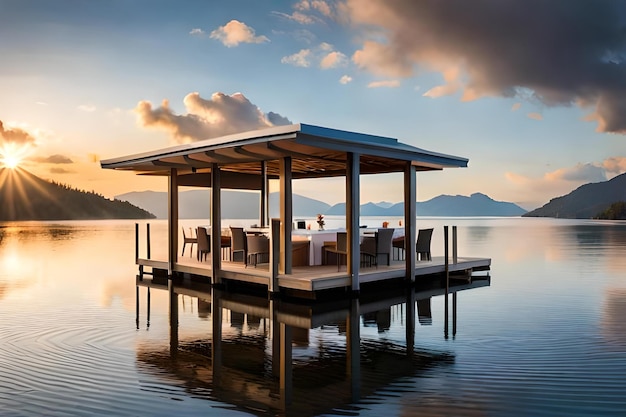This artwork depicts an ethereal outdoor scene with a serene lake at sunset or sunrise. In the middle of the still, blue water sits a gazebo-like structure, elevated on stilts. This open-air platform is minimalist in design, consisting merely of a roof, several pillars, and a spacious floor. At its center is an elegantly set dining area with a white table adorned with a vase of flowers and at least six upholstered grey chairs. The color palette is dominated by neutral hues—black, white, grey, and brown.

The tranquil setting is rendered against a backdrop of dark grey and purple mountains, with a range of smaller hills leading up to them. The sky above is a vivid blue, streaked with dark grey, orange, and red clouds illuminated by a glowing yellow sun that sits just above the horizon on the left side of the painting. This sun bathes the entire landscape in a warm light, enhancing the image's serene ambiance. No text or human activity disturb this peaceful scene, making it an idealized spot for quiet dining and contemplation amidst nature's beauty.